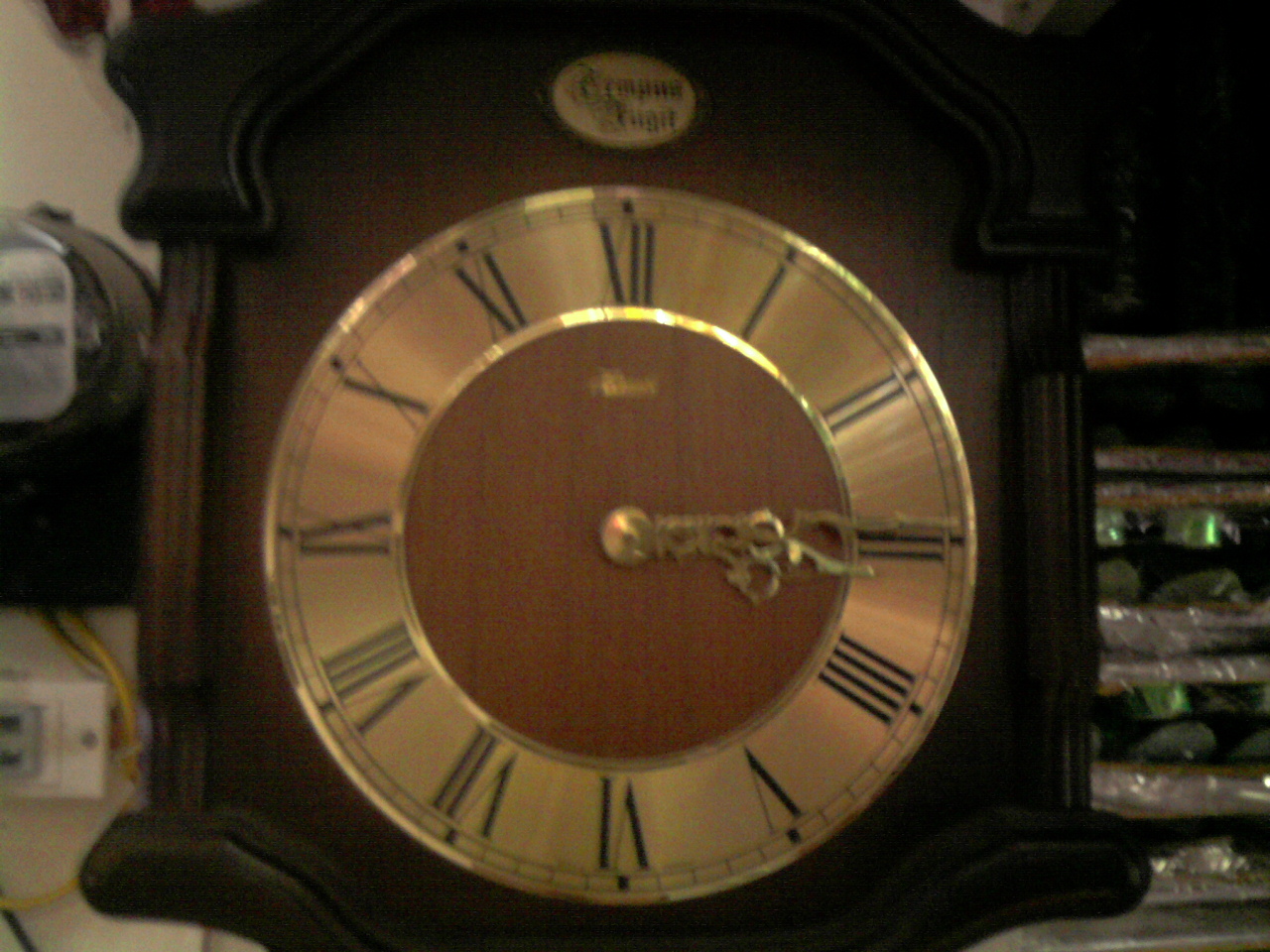This photograph is a slightly blurred, close-up image of the upper section of a dark wooden grandfather clock. The clock face is gold, adorned with Roman numerals in black from 12 to 11, and the minute and hour hands are also crafted from gold metal. Surrounding the clock face is a solid gold border that frames a darker, wood-grain interior. Above the clock face, there is an oval gold plaque with an inscription that is indistinct due to the blur. Similarly, beneath the Roman numeral 12, there's a name or brand in small gold letters that is unreadable. To the left of the clock, there is what appears to be an electric or gas meter mounted on a black base with a glass cover and a white label, against an off-white wall. Yellow and black wires extend from the meter, with the black wire running to the right of the clock. An outlet with a gray insert is also visible on the left side of the wall. In the background to the right of the clock, there's a dark brown object with silver details, whose exact nature is unclear. The bottom of the clock is cut off by the photograph's edge, leaving the base out of view.